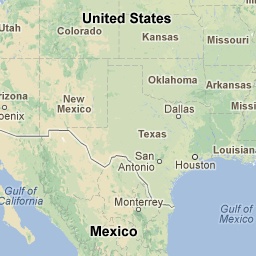This detailed map of the United States highlights the region extending from Mexico in the south to approximately Colorado and Kansas in the north. The westernmost boundaries of the map include Utah and Arizona, though the labels are slightly truncated. To the east, the map reaches as far as Missouri and Arkansas, with partial views of Mississippi and Louisiana. Central to the map is Texas, prominently displaying cities such as San Antonio and Houston. Both the Gulf of California to the west and the Gulf of Mexico to the east are visible, adding vivid blue expanses that contrast with the green and yellow hues representing the land. The names of the states and various geographic features are labeled in black, providing clear, readable points of reference amidst the colorful terrain.